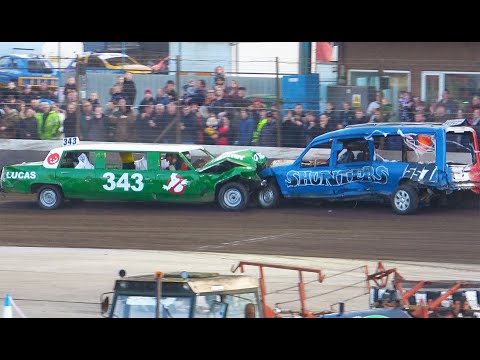In this dramatic screenshot from a video, two uniquely modified race cars have collided head-on during what appears to be a demolition derby event. The car on the left, an elongated green limousine, bears the number 343 prominently in white, alongside a Ghostbusters logo featuring a white ghost crossed out in red. The hood of the green car is dented and bent from the collision. The car on the right, a blue hearse-like vehicle, is labeled "Shunters" and displays the number 557. It sports a red, white, and blue color scheme and is also severely damaged from the impact. The scene is set on a brown dirt track, with several dozen onlookers visible behind a guarded wire fence, indicating a controlled and spectator-friendly environment. These spectators stand in front of a building structure, suggesting the event takes place in a designated venue. The image has black bars at the top and bottom, and the quality is somewhat subpar, making fine details slightly harder to discern.